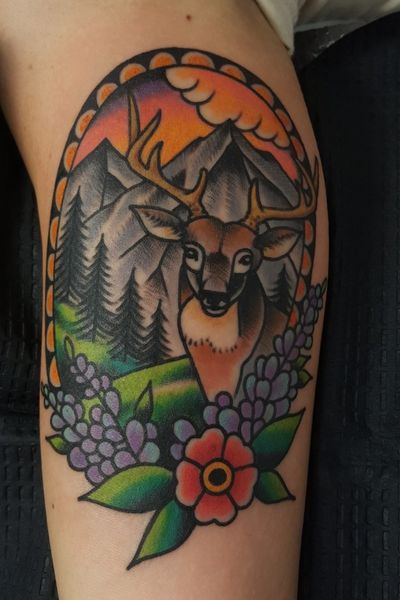This vertical rectangular image showcases a highly detailed tattoo on someone's arm, viewed from the side, with their shoulder bare and extending down to a couple of inches above the elbow. The tattoo features a vivid and elaborate scene: at its core is a majestic brown deer with tan antlers, positioned slightly towards the right. The deer's features include a black nose, brown eyes, and leaf-shaped ears with a white patch below them. Surrounding the deer is a natural setting with tall green trees and towering mountains in the background, enveloped in a mix of red, yellow, and orange hues that give a sense of a sunset or sunrise. Above the deer, there could be a mountain peak or possibly a native teepee, set against a sky where a cloud can be seen. The lower part of the tattoo includes green leaves and what appear to be berries or stones, along with a prominent red flower at the bottom. The background of the image is black, making the colorful artwork of the tattoo stand out even more vividly. The person appears to be wearing a black top, though their shoulder remains uncovered to fully display the intricate body art.